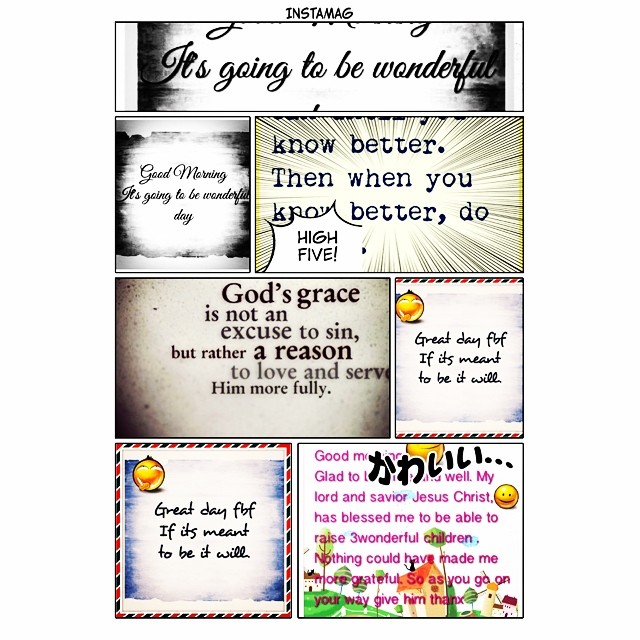The image is composed of a series of panels featuring motivational and inspirational text. At the top, the word "Instamag" appears in black letters. Below this header, the first panel spans the width of the image, showcasing black text on a white background that reads, "It's going to be wonderful."

The subsequent panels are arranged in a grid. The first column under the header includes:

1. **Panel 1:** A white background with black text stating, "Good morning. It's going to be a wonderful day."
2. **Panel 2:** A cream-colored background with radiating lines from the center and black text that says, "Know better. When you know better, do better." Additionally, a small white area within the panel contains the phrase "High five" in black text.

In the adjacent column, the panels are:

1. **Panel 3:** Features a brown background with black text that reads, "God's grace is not an excuse to sin, but rather a reason to love and serve Him more fully."
2. **Panel 4:** Displays a white background and gray text, alongside black text that reads, "A day off is meant to be, it will."
3. **Panel 5:** Contains a gradient background that fades from white to blue, with the words "Great day" in black text and "FBF, if it's meant to be, it will" in smaller font beneath it.

In the bottom right corner is a final panel with:

1. **Panel 6:** A white background featuring a cartoon village at the bottom. The panel carries a heartfelt message in purple text: "Good morning. Glad to see you're well. My Lord and Savior Jesus Christ has blessed me to be able to raise three wonderful children. Nothing could have made me more grateful. So as you go on your way, give Him thanks."

This detailed and vibrant collection of panels collectively delivers a message of positivity, faith, and gratitude.